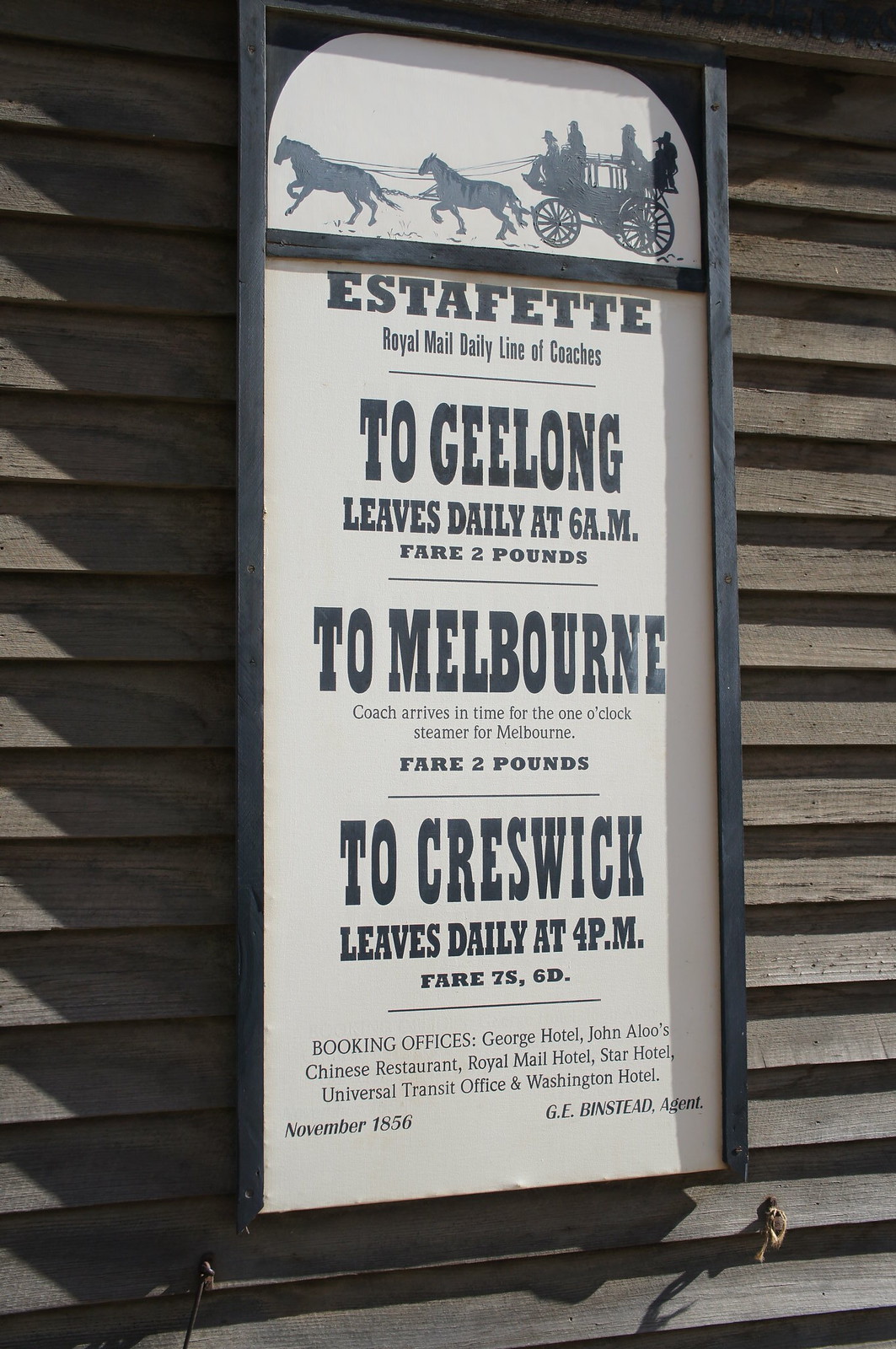This image captures an outdoor, daytime setting featuring an antique sign attached to a wooden slatted wall. The sign has a black border and prominently displays a detailed drawing of a stagecoach at the top, featuring two horses, a driver, and three passengers. Below the illustration, the text reads "Estafete Royal Mail daily line of coaches." The schedule informs readers that the coach to Geelong departs daily at 6 a.m. with a fare of two pounds, and the coach to Melbourne arrives in time for the one o'clock steamer, also with a fare of two pounds. Additionally, a coach to Creswick leaves daily at 4 p.m. with a fare of 7 shillings and 6 pence. The sign lists several booking offices: George Hotel, John Allu's Chinese Restaurant, Royal Mail Hotel, Star Hotel, Universal Transit Office, and Washington Hotel. The sign is dated November 1856 with G.E. Binstead as the agent. The vintage appearance of the sign and its content mark it as an obsolete piece, echoing a bygone era of stagecoach travel.